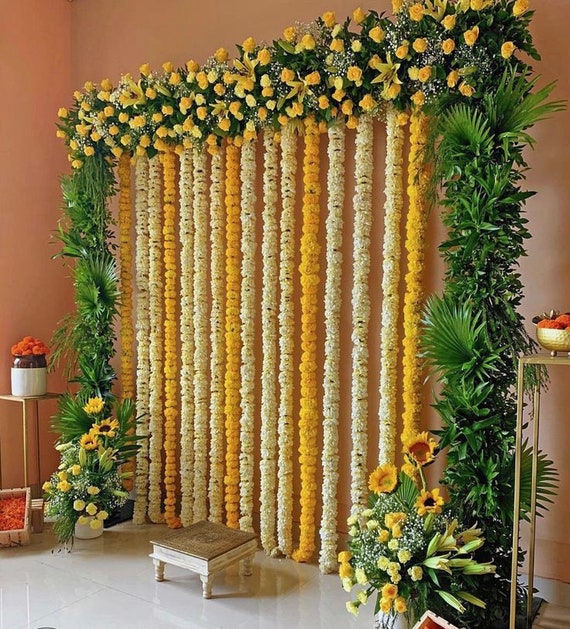The image showcases a decorative setup in a room with terracotta-colored walls, possibly intended for a celebration or a photograph backdrop. Central to the decoration is a rectangular arch formation adorned with an array of greenery and an assortment of yellow and white flowers, including roses, lilies, sunflowers, and baby's breath. The vertical sides of the arch are covered in lush green foliage, while the top horizontal element creatively integrates the green foliage with the colorful flowers. Long strings of yellow and white flowers cascade down from the top like leis, creating a visually striking curtain effect reminiscent of beaded doorways from the 70s. Below this floral arch, two tall golden tables are positioned on either side, each with its own floral arrangements. A small stool stands centrally beneath the archway, hinting at a possible focal point for future activities or a photo opportunity. The overall decor is intricately detailed, blending various shades of yellow and white flowers with the rich green foliage to form a captivating and celebratory ambience.